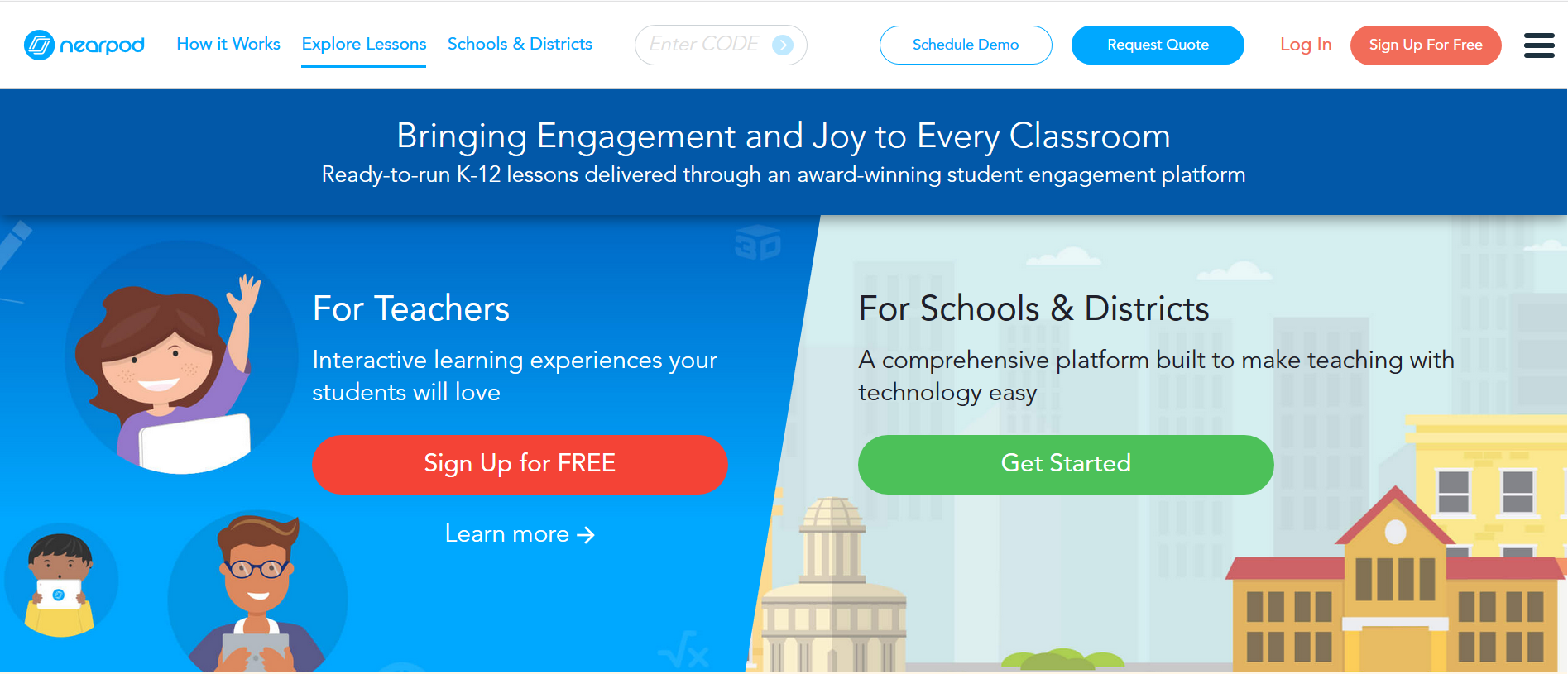The screenshot captures the homepage of the Nearpod website. Featured at the top, set against a white background, is a blue circular logo accompanied by the text "Nearpod." The main navigation menu displays options including "How it Works," "Explore Lessons," and "Schools and Districts." The "Explore Lessons" section is underlined, indicating the currently active page.

On the right side of the navigation bar, there are options to "Enter Code," "Schedule Demo," and "Request Quote," flanked by red-colored "Login" and "Sign Up for Free" buttons.

Beneath the navigation, a dark blue banner proclaims the platform's mission: "Bringing engagement and joy to every classroom." The banner elaborates with a subtitle that reads, "Ready-to-run K-12 lessons delivered through an award-winning student engagement platform."

The left section of the screen presents cartoon-style images depicting a student and several teachers. A heading beside these images states, "For Teachers: Interactive learning experiences your students will love," with options to "Sign Up for Free" or "Learn More."

The right section is dedicated to school districts, featuring a similar cartoonish design with images of schools. The heading announces, "A comprehensive platform built to make teaching with technology easy." Below this, a prominent green "Get Started" button invites users to take immediate action.

Overall, the page is visually engaging, using cartoon-style illustrations to convey a user-friendly and inviting atmosphere.